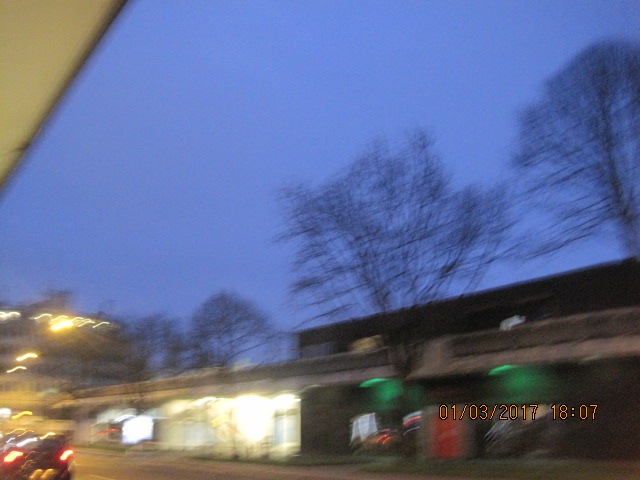The image captured on 01-03-2017 at 18:07 features a blurry, dusk-time street view in a suburban or city area, suggesting winter with bare trees in the background. The overcast sky has a blue tinge, indicating it is transitioning toward evening. Prominently, there's a multi-story apartment building on the back left with shielded lights underneath, possibly illuminating a shop or a structure below it. A car with its taillights on is traveling along the street, which is lined with a mixed landscape—bare trees, probable shops on the other side, a white fence, and what appears to be a dirt road. The timestamp of the surveillance footage is clearly marked in yellow at the bottom right of the image.